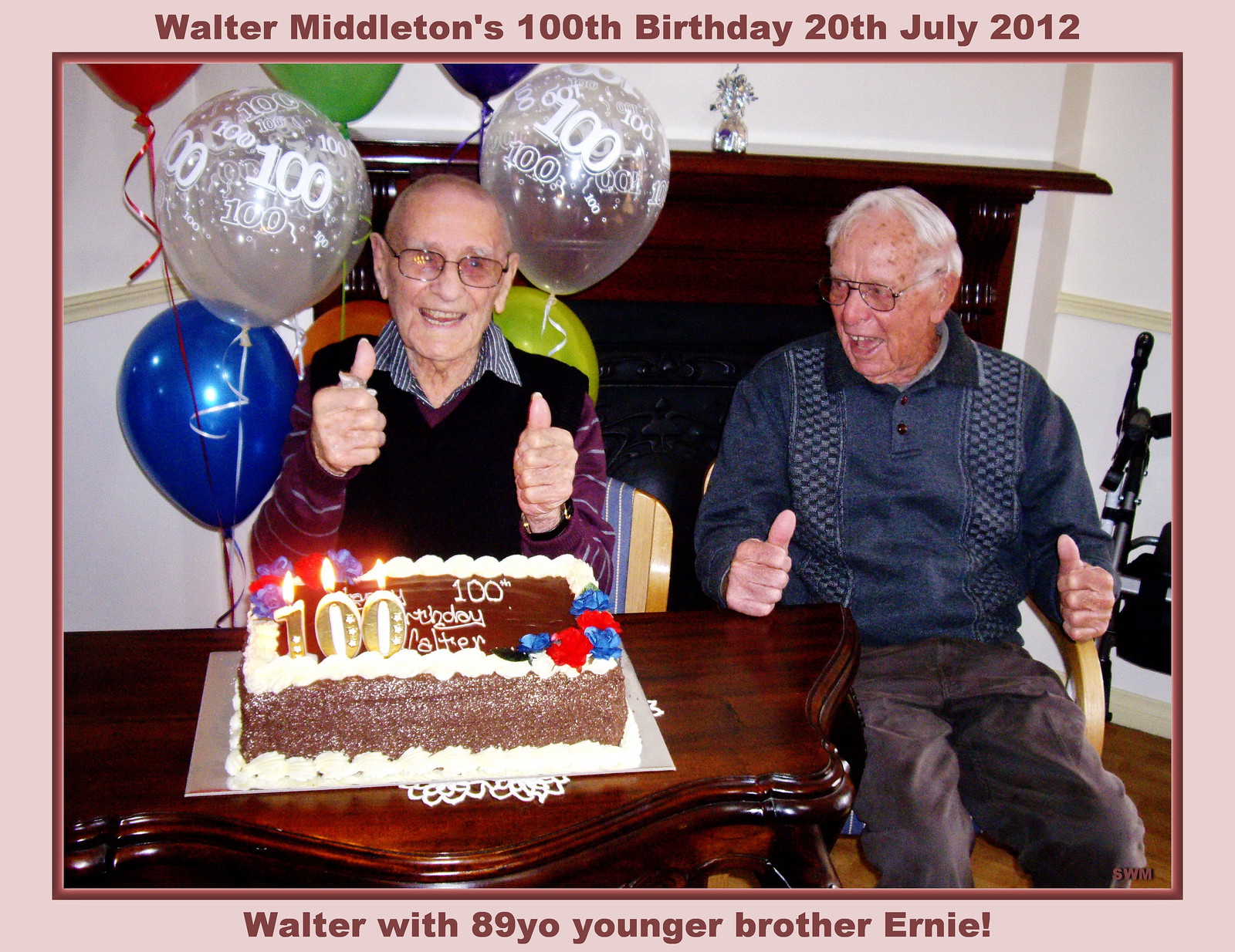This digital photograph captures a heartfelt moment during Walter Middleton's 100th birthday celebration on July 20th, 2012. The image prominently features two gentlemen: Walter Middleton on the left, and his younger brother Ernie, aged 89, seated next to him. Both men are joyfully giving a thumbs-up in front of a beautifully decorated birthday cake, which sits on an ornate table. The cake, featuring cream-colored icing with chocolate brown layers and adorned with vibrant blue and red rosettes at its corners, has candles forming the number '100' that are lit. Surrounding Walter are festive '100' balloons, adding a celebratory ambiance to the scene. The room's setting includes a cozy fireplace, two chairs, and a well-lit interior that brings warmth and charm to the entire composition. The top of the image reads "Walter Middleton's 100th birthday, 20th of July 2012," while the bottom identifies the brothers with the caption "Walter with 89-year-old younger brother Ernie." The array of colors—white, blue, green, red, black, brown, gray, and orange—contribute to the joyful and vibrant atmosphere.